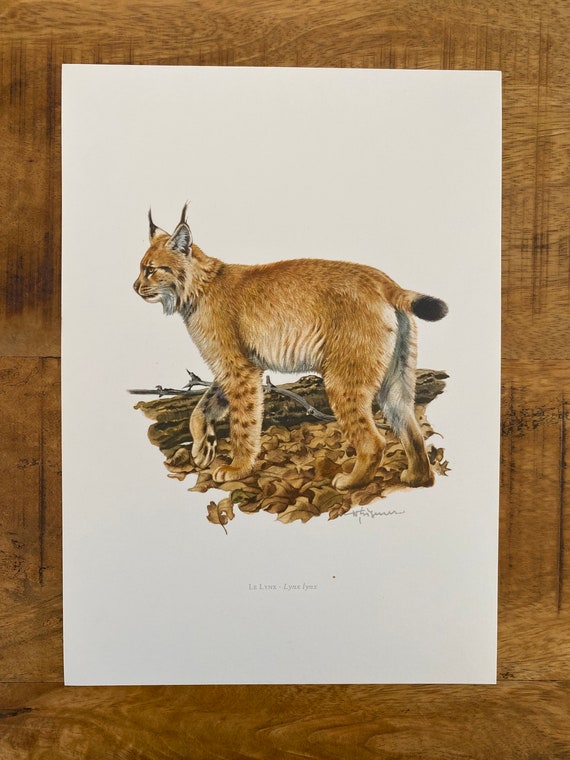The painting is exquisitely detailed and framed in a wide wooden frame featuring a mix of light, dark, and black wood grain. It's mounted on off-white paper set against a wood-textured background. At the center is a depiction of a lynx with a light brown, fluffy coat and distinctive characteristics such as white fur on its belly, rear, and breast. It also has prominent black tufts at the tips of its pointy ears and golden eyes, although it's facing to the left. The lynx has spots on its legs – polka dots on the front and stripes on the back – and white whiskers add to its realistic charm. Its right front paw is raised, revealing its white underside, and it has a short bobtail with a black tip. The scene is set in a natural woodland environment, with the lynx standing on brown leaves and a downed tree branch or log in the background. At the bottom of the piece, the signature reads 'le lynx – lynx lynx,' though the artist's name is not clearly legible.